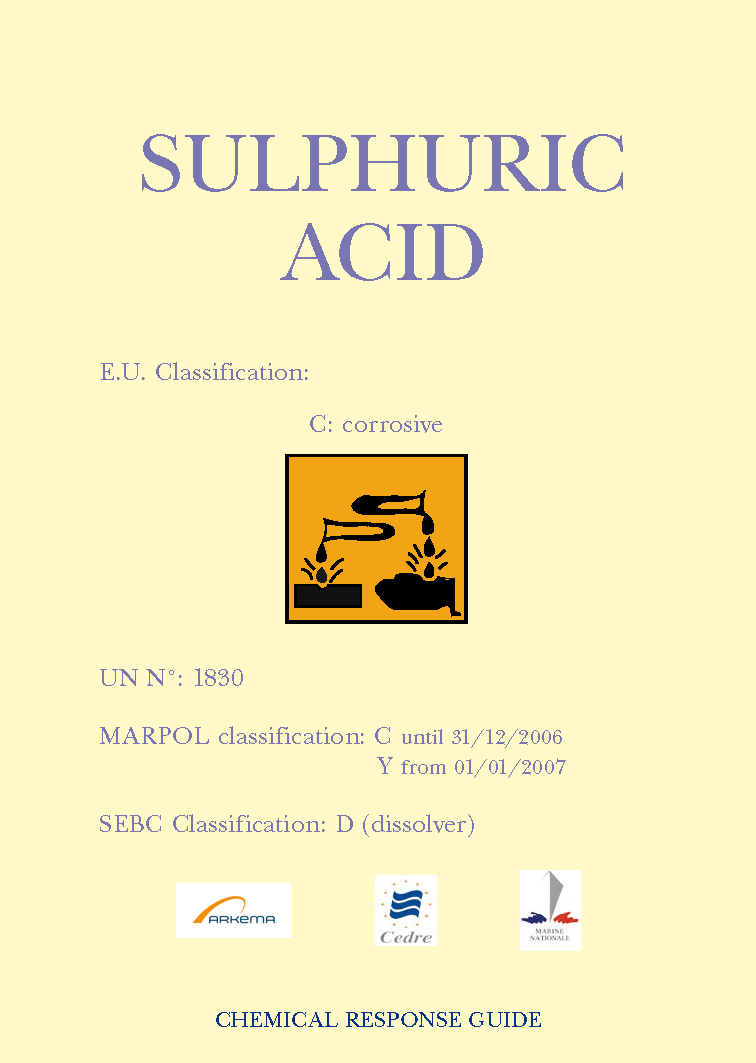This detailed poster is designed to inform about sulfuric acid, featuring a pale yellow background with medium purple text across the top that reads "Sulfuric Acid." The poster details its EU Classification as C (Corrosive) and includes the identifier UN N° 1830. The MARPOL Classification is noted as C until 31/12/2006 and Y from 01/01/2007, while the SEBC Classification is listed as D (Dissolver). Below these details, there's an image in dark yellow illustrating various chemicals and their reactions. The poster also includes three small, colorful icons: a blue wavy flag, an orange hook-like symbol, and a 3D triangle with blue and red sides. At the bottom, it states "Chemical Response Guide," potentially indicating its usage in workplaces to warn or inform employees about handling sulfuric acid.